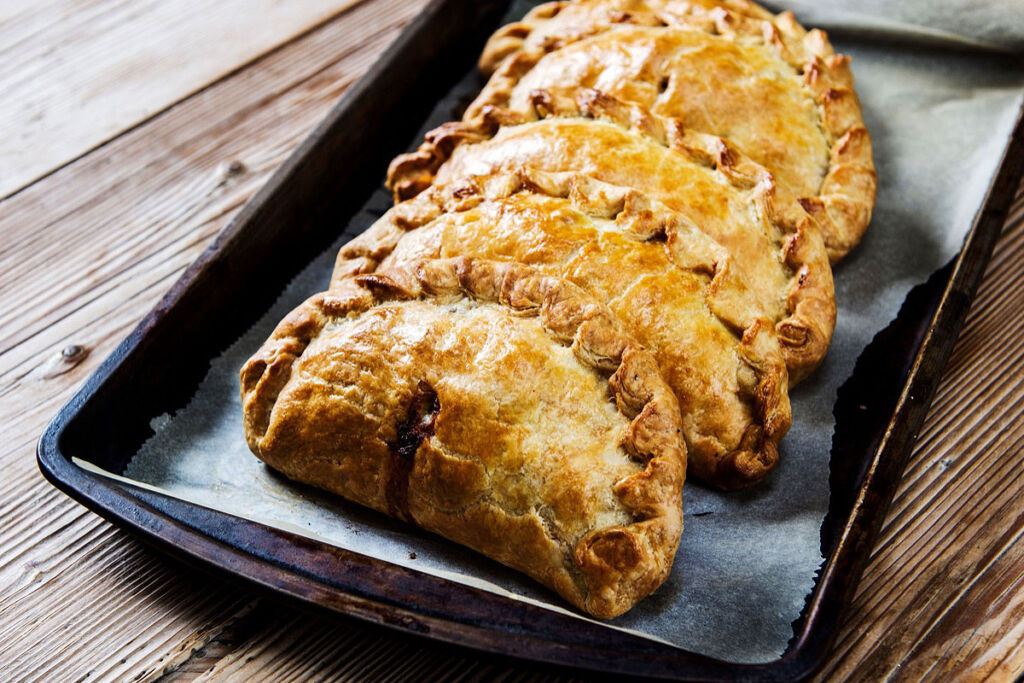This photograph captures a rustic scene of freshly baked pastries, possibly meat pies or fruit-filled pockets, presented on a well-seasoned, blackened baking sheet resting atop a wooden table. The baking sheet is lined with parchment paper, ensuring the pastries don’t stick. There are four golden brown, crescent-shaped pastries, each crimped along the edges to keep the filling contained. Although the exact filling is indeterminate, it could range from a rich jelly to a savory meat mixture. The pastry edges are pinched, and some have a small slice in the center. The pastries exhibit a shiny, flaky texture, suggesting they were brushed with an egg wash before baking, adding to their appetizing appearance. The pastries are nestled closely together, reminiscent of tacos in a box, highlighting their homey and delectable charm.